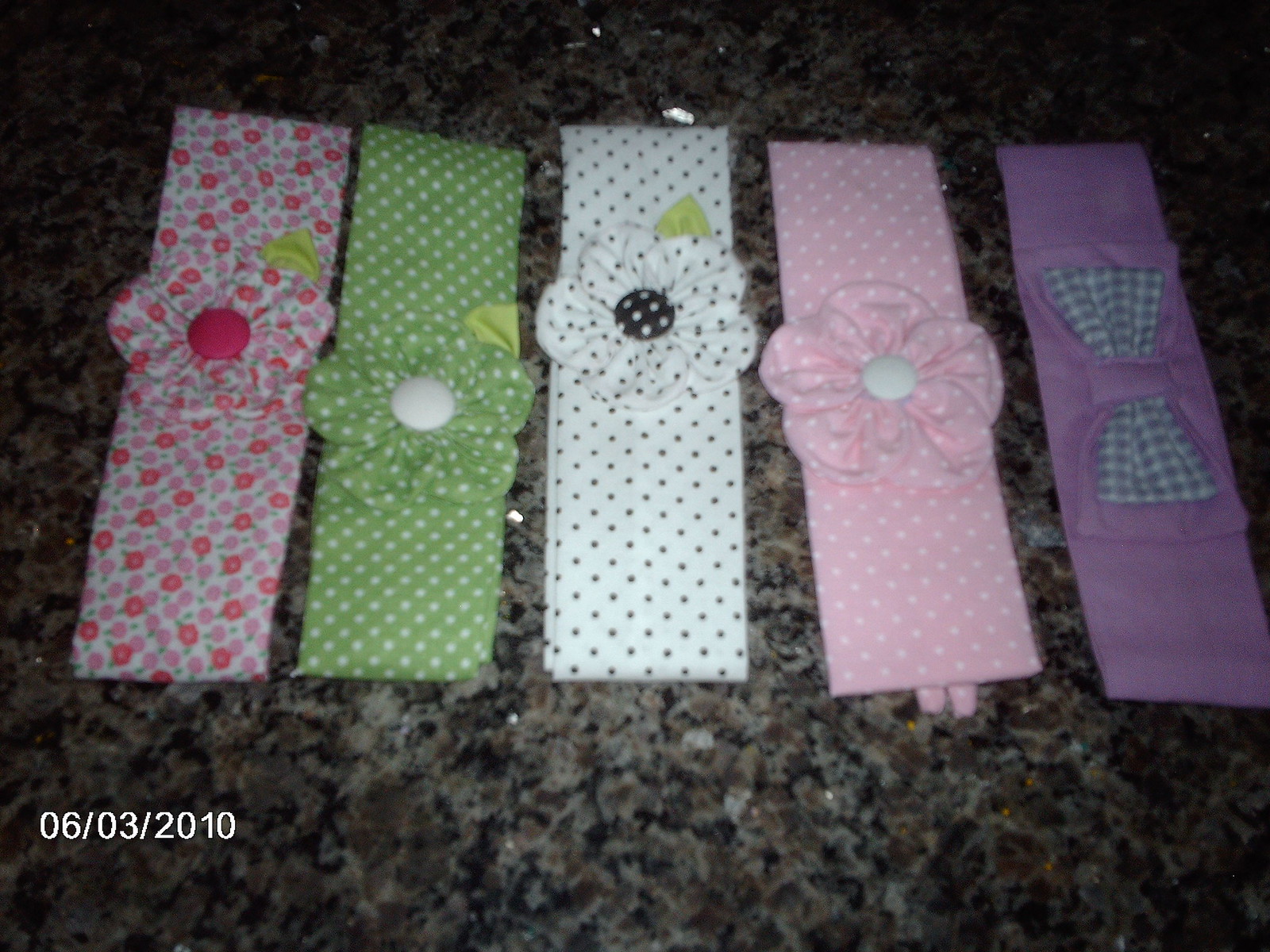This photograph, taken on 06-03-2010, showcases an array of colorful and patterned headbands neatly arranged on a dark marble surface, most likely inside someone's house. The vibrant and cheerful headbands, which appear to be designed for little girls, feature a variety of patterns and decorations. Starting from the left, there is a pink headband adorned with red, yellow, and pink floral patterns and a green leaf. Next is a green headband with white polka dots and a floral bow that includes green leaf details. The center headband is white with black polka dots and a floral bow, also accented with a green leaf. Following that, there is another pink headband with white polka dots and a floral bow. The final headband on the right is a plain purple band with a bow that has a black and white checkered interior pattern. Despite the photograph's overall dark tone, the headbands' vibrant colors of pink, light green, and light purple, along with their floral and polka dot patterns, stand out vividly against the dark marble surface.